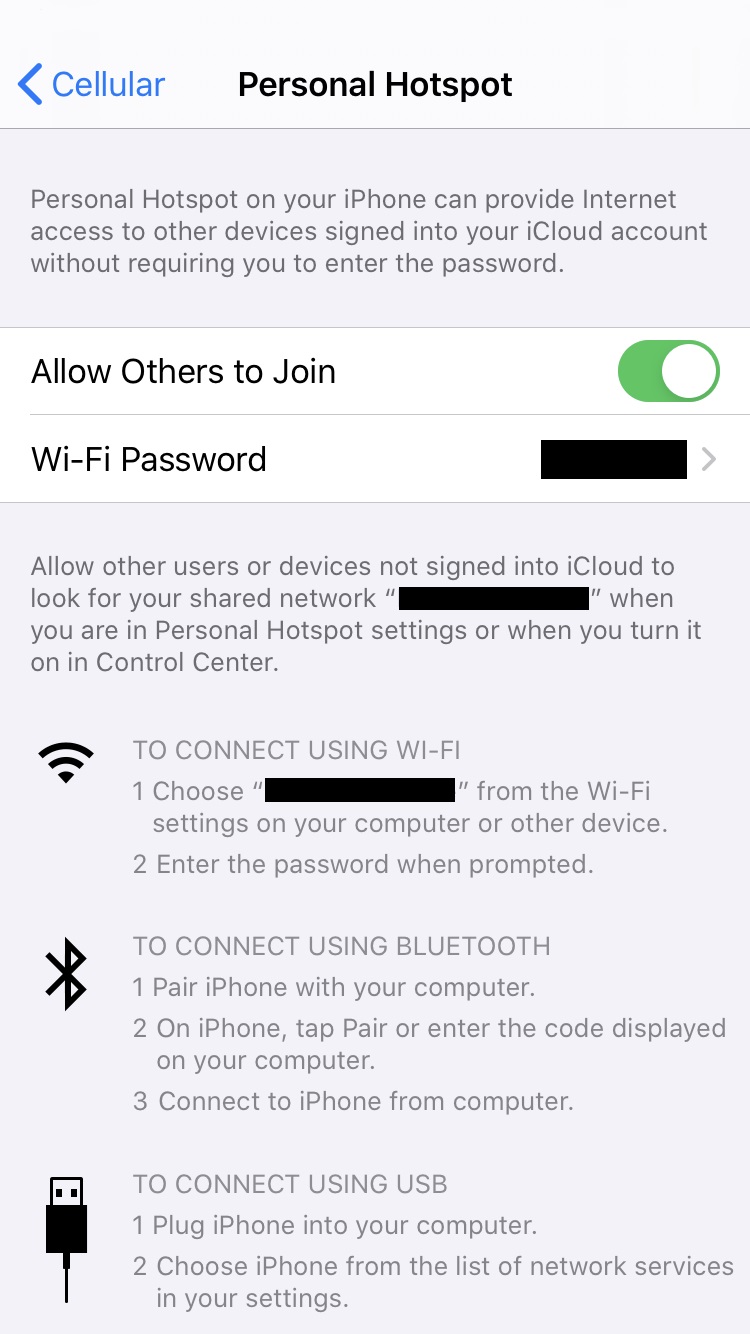This screenshot features a light gray background and displays a section from an iPhone's settings. 

In the top-left corner, there is a blue arrow pointing to the left, resembling a less-than symbol, next to the word "Cellular" in blue. Adjacent to this, "Personal Hotspot" is written in black.

Directly below, there is a darker gray informational box stating: "Personal Hotspot on your iPhone can provide internet access to other devices signed into your iCloud account without requiring you to enter the password."

Beneath this, a section with a white background reads "Allow Others to Join." A toggle switch on the right is activated, shifted to the right and displayed in green.

Following this, a thin horizontal line separates the sections. 

Next, it reads "Wi-Fi Password," which is partially obscured by a black box. To the right of this, there's a greater-than symbol indicating additional options.

Below that, a larger darker gray text box appears. It explains: "Allow other users or devices not signed into iCloud to look for your shared network." The subsequent text is blacked-out, indicating hidden options or instructions. At the bottom, it says "When you are in Personal Hotspot settings or when you turn it on in Control Center," followed by Wi-Fi signal instructions and the phrase "To connect using Wi-Fi."

This detailed description highlights the intricate settings available for managing a personal hotspot on an iPhone.